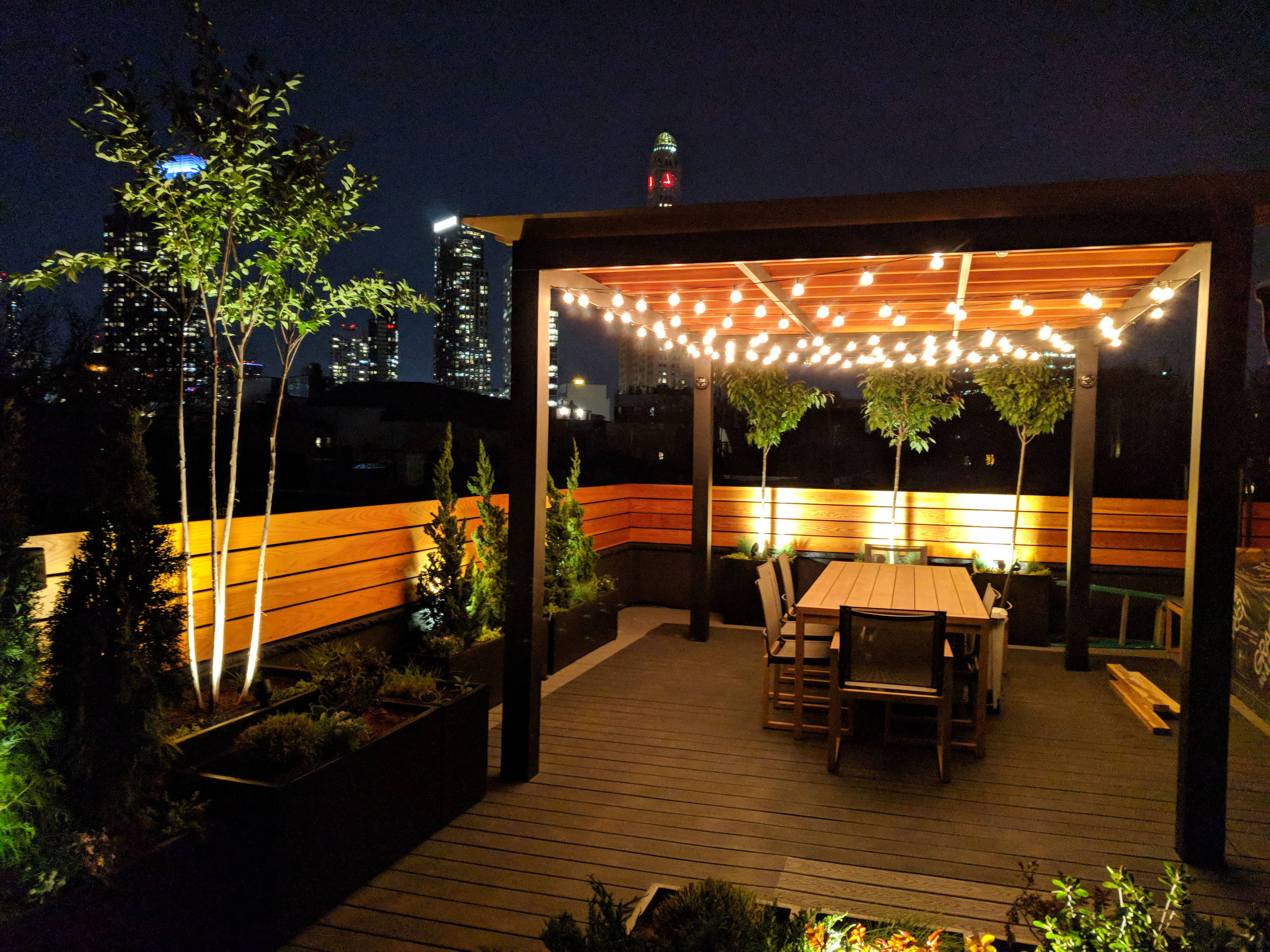The photograph showcases a dramatically lit, upscale outdoor dining area, likely part of a restaurant or hotel terrace. The central focus is a wooden gazebo with four pillars and a roof, under which hangs a series of small white string lights, creating an elegant ambiance reminiscent of a wedding setup. Beneath the gazebo is a large dining table surrounded by eight chairs, all set on a raw, untreated wooden deck. The fencing and siding are also made of wood, specifically cedar, adding to the rustic yet sophisticated atmosphere. The perimeter and fence are adorned with dramatic lighting, illuminating the lush green vegetation, including trees, shrubs, and other plants. In the background, the night sky reveals a distant cityscape with large, illuminated skyscrapers that suggest the setting might be in San Antonio, Texas. The overall setting is empty of people, highlighting the serene and inviting nature of the space.